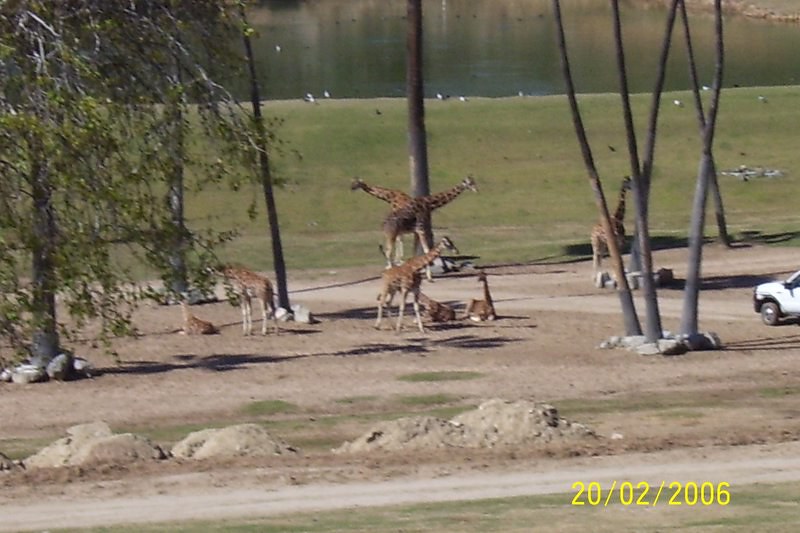This detailed photograph, likely taken with a low-quality digital camera in 2006, depicts a zoo or drive-thru safari exhibit featuring several giraffes. The image, timestamped "20-02-2006" in yellow font at the bottom right corner, showcases the diverse landscape of the setting. In the upper portion of the photo, there is a brown freshwater pond bordered by a green, grassy field where tiny white dots, possibly birds, are visible. At the intersection of the grassy expanse and a sandy, dirt-laden area, there are about nine or ten trees sprouting up. Scattered across the foreground are seven or eight giraffes, with some milling around and two situated on the ground. Also visible in the image is a white vehicle, likely a zoo truck, parked to the side near piles of dirt, reinforcing the zoo or safari environment.